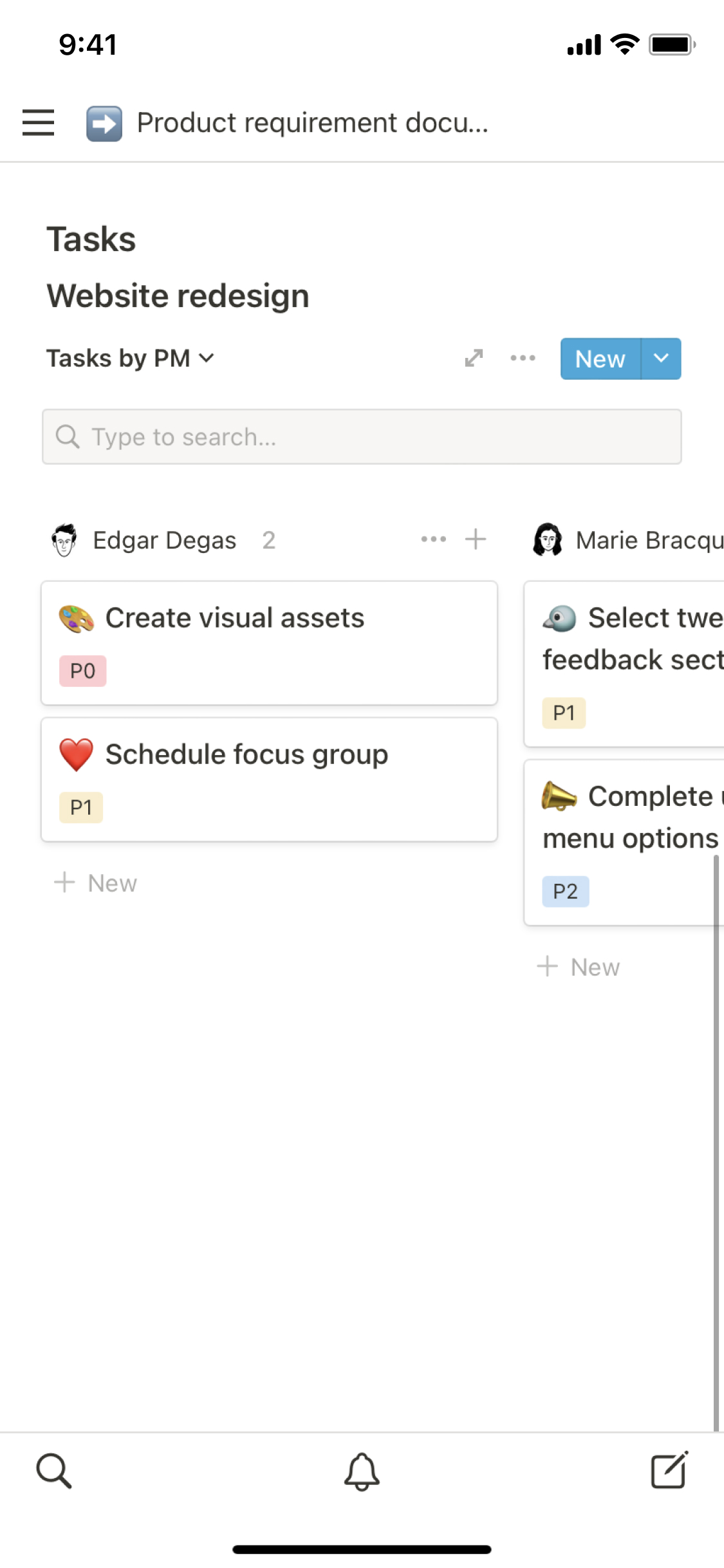Screenshot of a cell phone displaying a task management application:

At the top of the screen, the time is shown as "9:41 a.m." on the left side, while on the right, there are icons indicating signal strength, Wi-Fi strength, and battery status. The background is entirely white. Just below this status bar, on the left, there are three horizontal lines representing a menu. Next to this is a grey block containing a right arrow, followed by a truncated file name, "Product Requirement Docu...".

In a white block below this, bold black text reads "Tasks: Website Redesign", with a sub-header "Tasks by 9 p.m." To the right of "9 p.m.," there are three vertical dots indicating more options, and a blue button labeled "New" with a drop-down arrow.

Further down is a light gray search bar with a magnifying glass icon and the prompt text "Type to search". Below this section, there are various tasks listed with associated visual elements:

1. "Edgar Degas" accompanied by a drawing of a man’s head.
2. "Create visual assets" next to an illustrative image.
3. "Schedule focus group" with a heart icon.

In the right-hand column, there is a cutoff image of a woman and the text "Marie Braque". Below this, "Select tweets for feedback" with a bird's head icon, and "Complete something" near menu options.

At the bottom of the screen are navigation icons: a magnifying glass for search on the bottom left, a bell for setting reminders in the center, and a square with a pen diagonally in the top right corner representing the option to add notes.